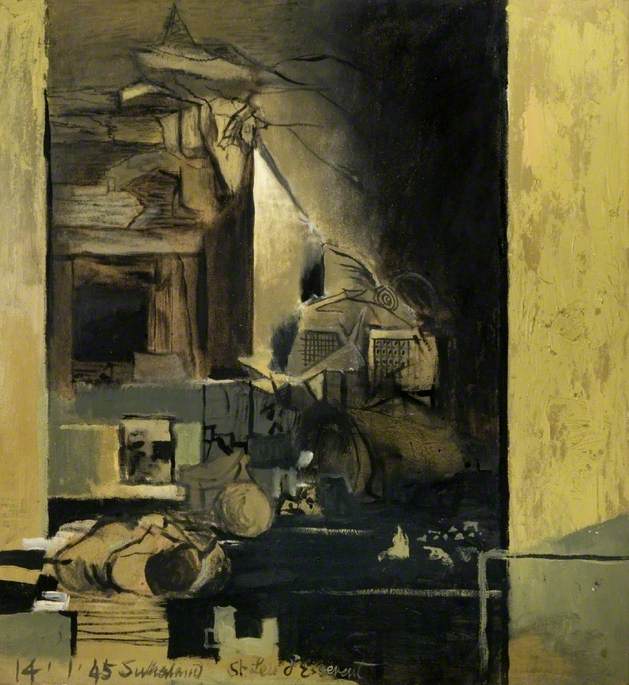This painting is an abstract and dark sketched composition, predominantly featuring shades of dull yellowish tan and black with subtle accents of white. The image seems to depict the inside of a dilapidated building or tunnel, possibly made of wood, with a cracked ceiling and various indistinguishable objects scattered across the floor. The right side displays vertical tan stripes resembling a door frame or entrance, while the left side also features similar tan hues. The central area of the painting is consumed by dark, almost black tones, interspersed with narrow, precise lines and shapes that suggest a coal mine shaft or cave-like structure. At the bottom left-hand corner of the painting, there is a handwritten signature and the cryptic numbers "14145," though the exact words are hard to decipher. The overall atmosphere of the artwork is somber and mysterious, with various elements contributing to its enigmatic and fragmented appearance.